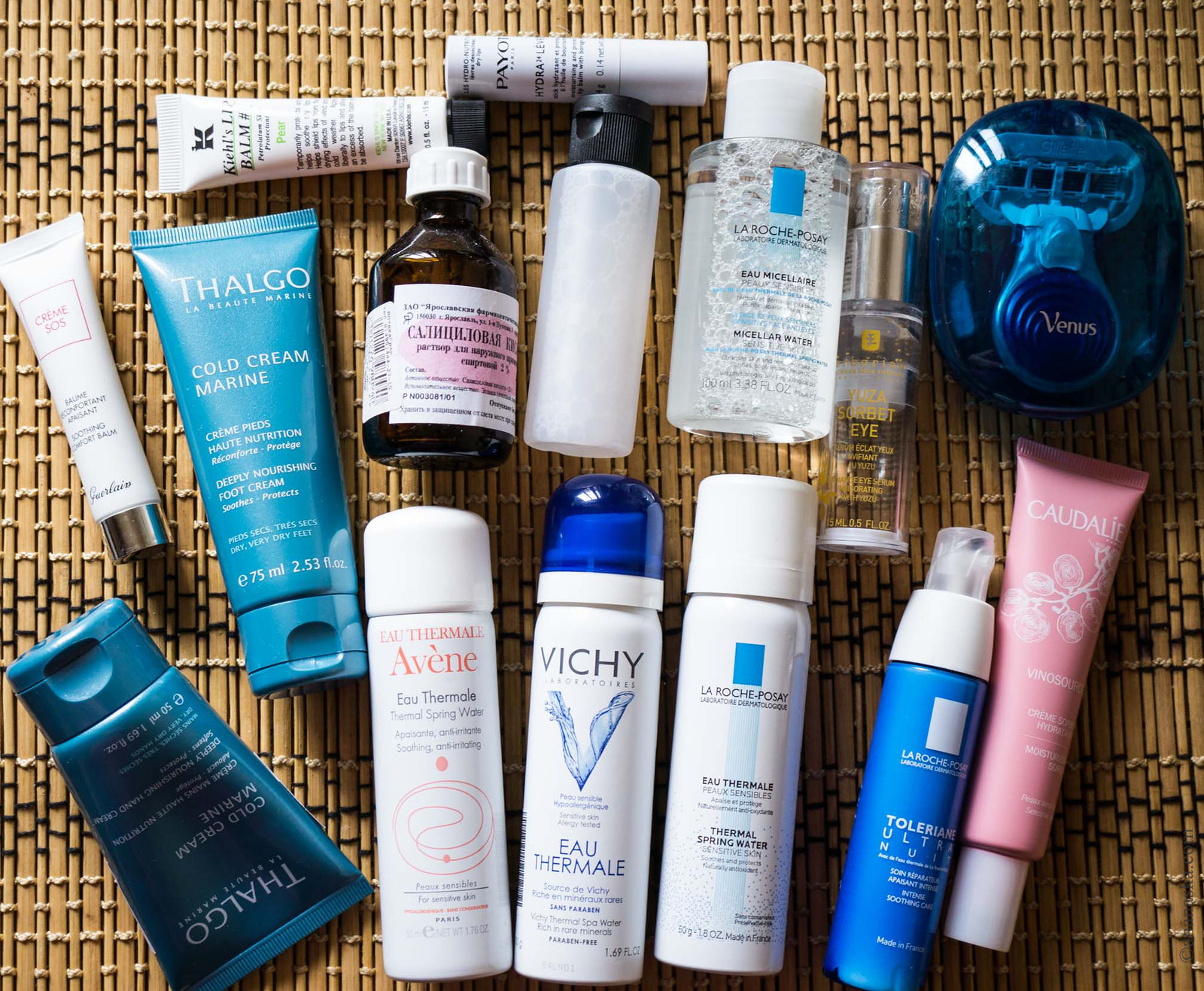The image showcases an artfully arranged assortment of beauty products placed on what appears to be a brown, wooden placemat. The careful placement of these items suggests the photograph was staged for promotional or aesthetic purposes. In the upper right corner, a Venus razor blade is visible, encased in an oval-shaped, transparent blue container marked with the "Venus" logo. Adjacent to the razor, there are various liquid beauty products in bottles, including an eye gel, which is often mistaken for an eye cream, and a makeup remover housed in a squirt bottle. The collection also features two distinct lip balms, along with a blue and silver cold cream from Thalgo in a squirt bottle. Towards the bottom of the image, a variety of facial sprays are displayed: one is a white and peach-colored spring water spray bottle for the face, and another is a competitive brand's spring water spray in a blue and white container. The overall presentation is aesthetically organized, highlighting the diversity and functionality of the beauty products.